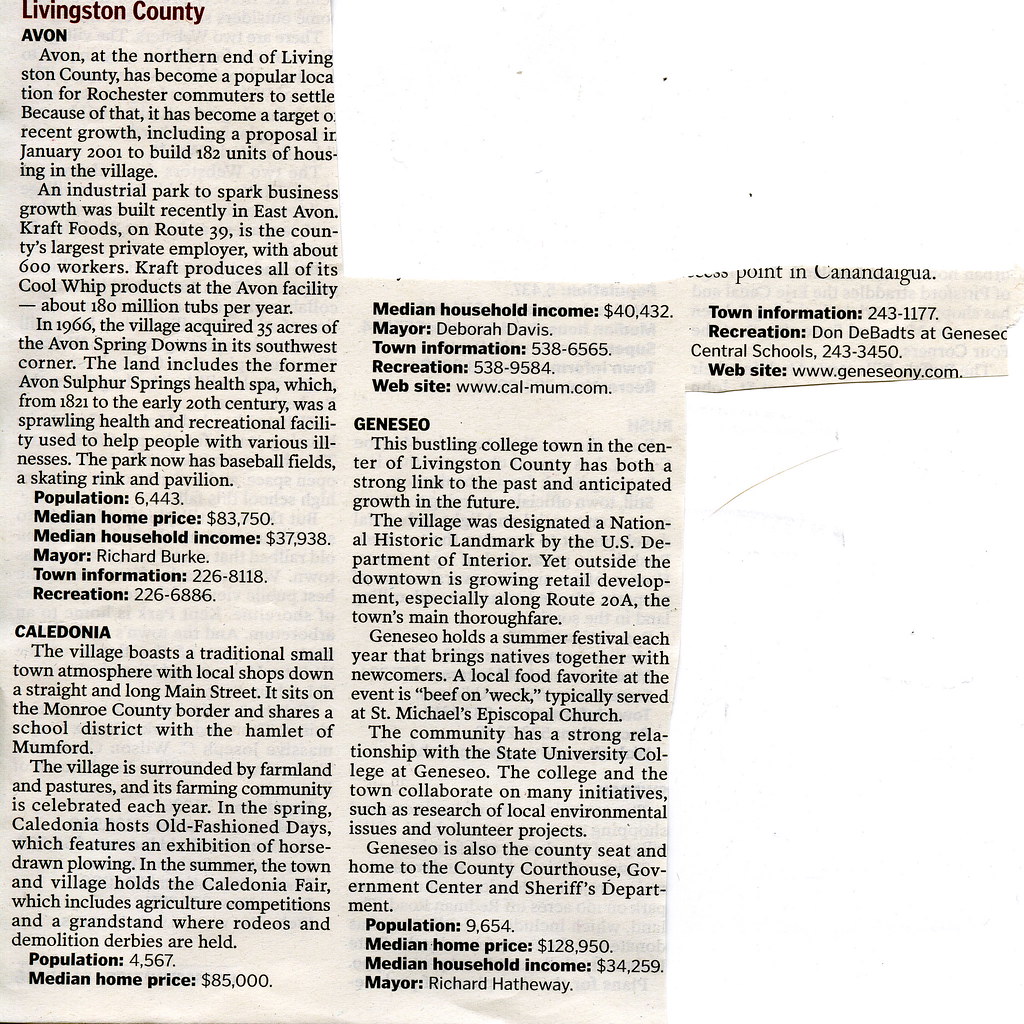The image is a detailed excerpt from an old newspaper showcasing various places within Livingston County, specifically focusing on Avon, Caledonia, and Geneseo. The newspaper's text is printed on a background of white, tan, maroon, and black, with the clipping occupying most of the visual space.

**Livingston County:**

- **Avon:** Positioned at the northern end, Avon is a favored destination for Rochester commuters and has experienced significant growth. Highlights include a proposed 182-unit housing development in January 2001, an industrial park in East Avon fostering business growth, and Kraft Foods on Route 39, the largest private employer in the county, with about 600 workers producing all Colwood products. Population: 6,443. Median Home Price: $83,750.

- **Caledonia:** A village that retains a traditional small-town atmosphere, featuring local shops and a charming Main Street. The area description spans two paragraphs, providing additional community information. Population: 4,567. Median Home Price: $85,000.

- **Geneseo:** A vibrant college town located in the center of the county, known for its balance between historical significance and future growth. The town's description includes five paragraphs detailing its bustling nature and academic environment. Population: 9,654.

Additionally, the text mentions categories such as median household income, mayor, town information, recreation, and website links for each town, although specific details for these categories are not fully outlined in the provided fragments.